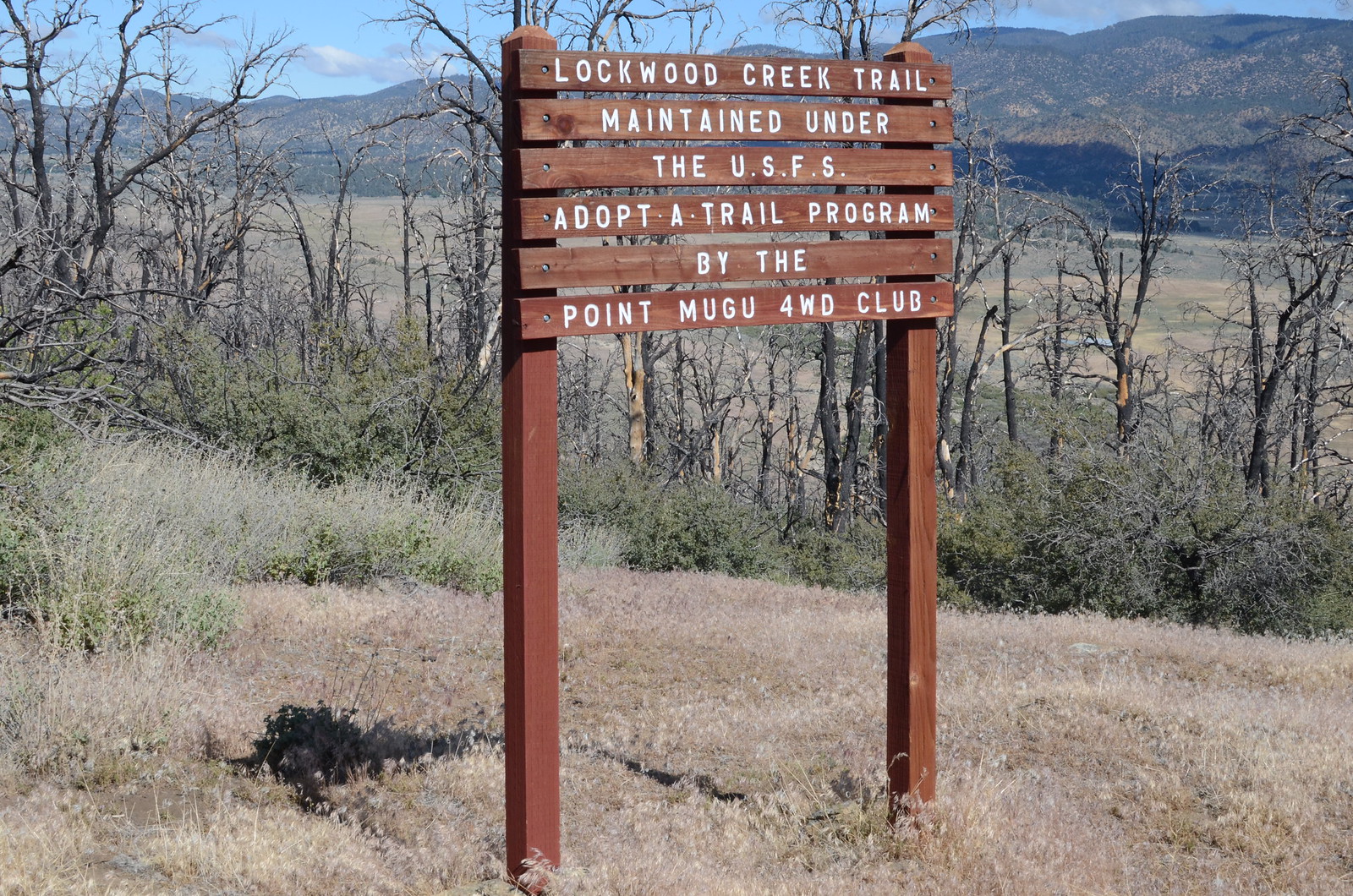The image features a rustic wooden sign comprised of six horizontal strips of wood with white, all-caps lettering that reads, "Lockwood Creek Trail, maintained under the USFS Adopt-A-Trail Program by the Point Mugu 4WD Club." The sign is supported by two sturdy 4x4 posts, planted firmly into the ground which is covered with brown, dried grass. A shadow of the sign is visible on the ground, indicating a sunny day. The backdrop includes leafless trees, scattered bushes, and shrubs, leading to a large field and mountainous terrain in the far distance. Above, the sky is a clear blue with some clouds, enhancing the serene, natural setting of this trail marker.